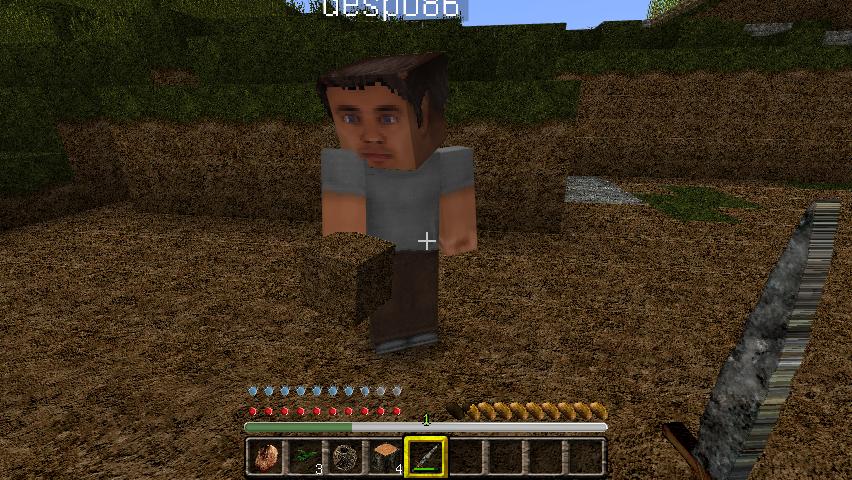In this image, we see a unique blend of realism and pixelation within a Minecraft world. The focal point is a Minecraft character with an unusually realistic face, seemingly transferred from a digital photograph. The character's head maintains Minecraft's blocky structure, but the face is rendered with impressive detail, depicting a man with light brown hair and a slightly tanned complexion, possibly Hispanic. This man is carrying a block which appears to be a common ground block, but its texture is indeterminate. The perspective is in first-person view, showing the main character holding a stone sword as if preparing to interact with or confront the approaching character. The juxtaposition of the hyper-realistic facial detail against the traditional Minecraft environment creates a visually intriguing and slightly surreal scene.